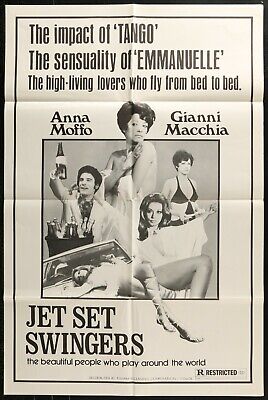This appears to be a vintage movie poster, aged and worn with visible fold marks. The poster features a black and white color scheme and is framed with a thin black border around the edge. At the top, in bold black text, it reads: "The Impact of Tango, The Sensuality of Emmanuel, The High Living Lovers Who Fly From Bed to Bed." The names Anna Moffo and Gianni Macchia, spelled M-A-C-C-H-I-A, are prominently displayed near the top and to the upper right of a central square photograph.

The central image showcases multiple intriguing elements: a man with dark, curly hair resembling an Afro, dressed in a suit and holding a champagne or wine bottle with a bucket of bottles beside him; a nearly nude woman attempting to cover herself with a dress and her arm; another woman in a bikini with her hair cut short to her ears; and a woman with long, wavy hair in a white gown reclining, with her legs exposed. Part of the image also appears to show a duplicate of the reclining woman, lying atop a car hood.

Below the photograph, the text continues in bold: "Jet Set Swingers, the beautiful people who play around the world." In the bottom right corner, the final statement reads: "Are Restricted," adding a sense of exclusivity or limitation to the theme. The overall impression is one of glamor and high society, captured in an evocative portrayal typical of old movie posters from the 1950s and 60s.